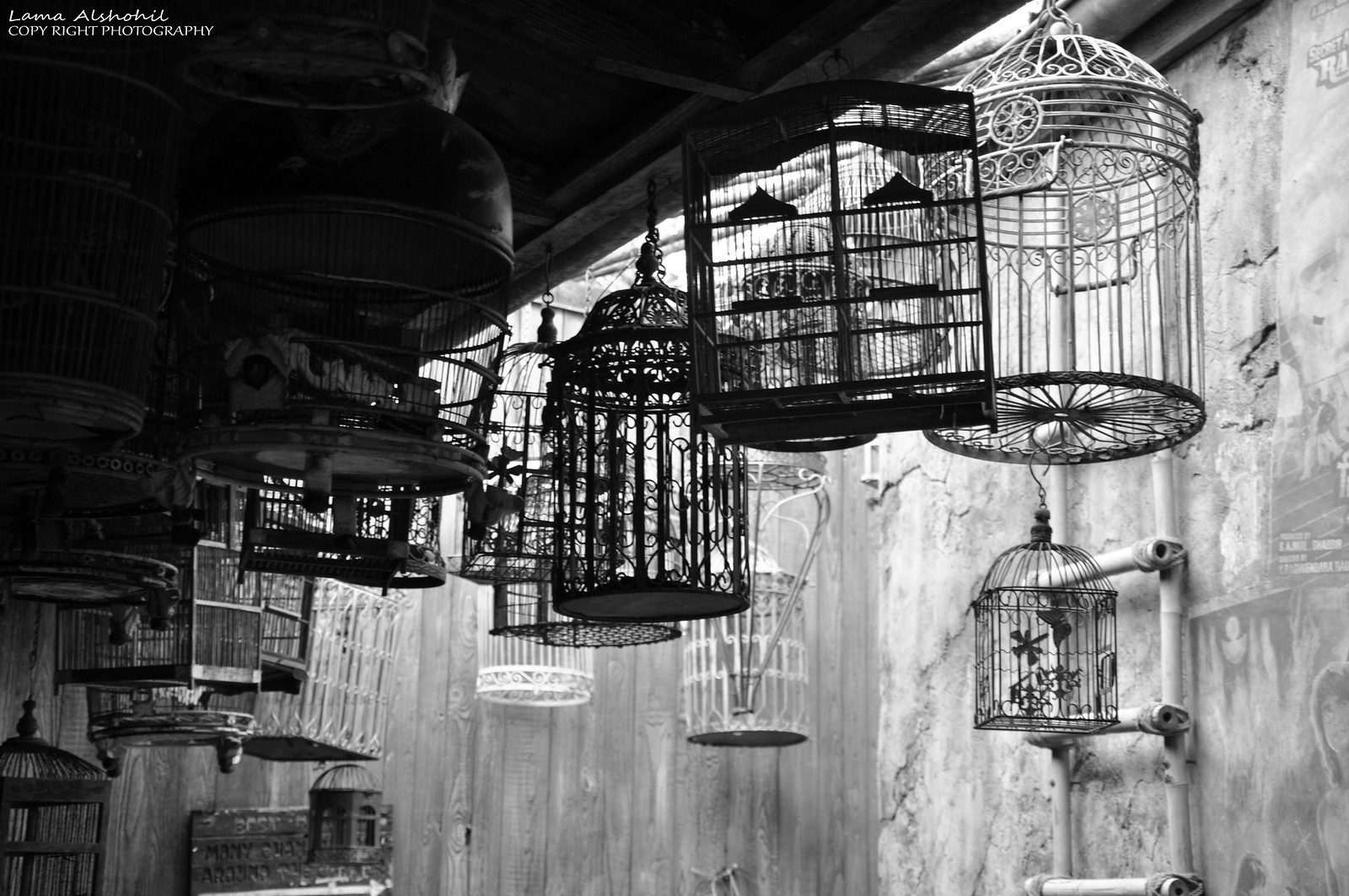The black and white image captures an array of birdcages hanging under an awning that spans the upper left side of the photograph. The awning shelters the intricately designed cages, casting shadows that add to the composition's depth. In the upper left corner, cursive text reads "Lama Alshohil," with "COPYRIGHT PHOTOGRAPHY" inscribed in white uppercase letters below. The cages themselves vary in shape and design, predominantly round with ornate lids, yet a notable rectangular cage occupies the upper center of the image. Outside the awning, a textured stone wall forms the backdrop, adding a rustic feel to the scene. To the right, a white ladder ascends the stone wall, partially obscured behind the hanging cages. The interplay of light and shadow varies across the composition, accentuating the different tonal qualities of the grouped birdcages.